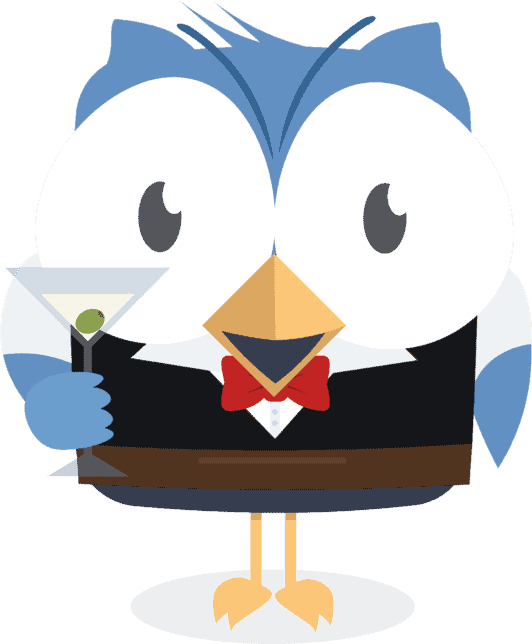This image depicts a comical and charming caricature of a blue owl prominently positioned against a white background. The owl is characterized by its large, round eyes with black crescent-shaped pupils and a vivid yellow beak, which is highlighted by its open, smiling expression. Perched in its right hand is a clear martini glass containing a single green olive. The owl is dressed in a stylish tuxedo ensemble, complete with a red bow tie, a white shirt adorned with two buttons, a black jacket, a brown belt, and dark brown pants. The bottom of the creature is rounded off by an oval color circle, seamlessly blending the brown and blue hues of its finely detailed feathering. This whimsical illustration captures a lighthearted yet sophisticated party vibe, combining intricate attire with playful features like the half-moon eyes and vibrant color palette.